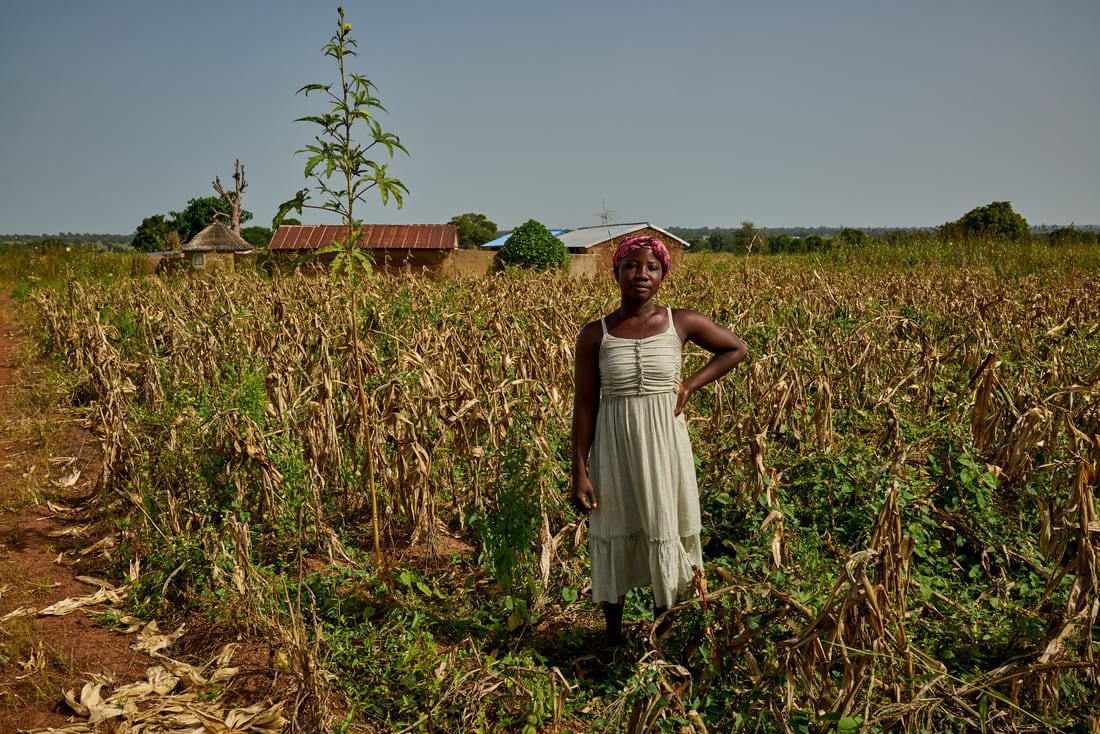This photograph features a young, dark-skinned woman standing prominently in the center of the image. She is wearing a sleeveless white dress made of light cotton fabric that extends down to her shins, fitting more snugly around the chest. The dress has delicate white straps. On her head, she has a pink or red bandana that keeps her hair tied up. Her left hand is confidently placed on her hip with her elbow pointing outward, while her right arm rests straight down by her side. 

The backdrop reveals a desolate field with old, possibly harvested stalks that look similar to sugar cane or corn, now mostly dried and brown. There are remnants of green, suggesting it might be late summer or a result of a heat wave. In the hazy background, several primitive-looking structures are visible, including a round home and a longer building with reddish roof tiles. Additional structures can be seen, one with a white roof and another with a blue roof, all under a gray sky, adding to the rustic and somewhat barren ambience of the scene.